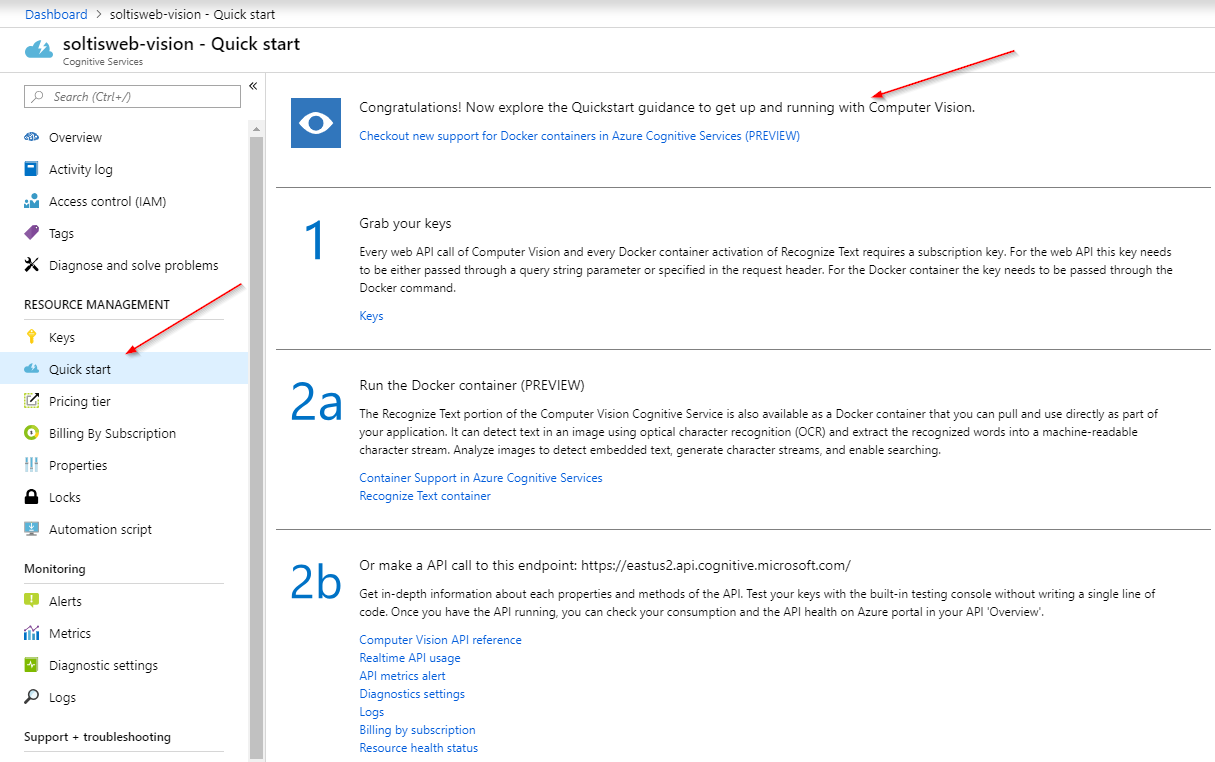### Caption for the Image:

The image showcases a user interface, likely of a website or application, against a clean white background. In the upper left-hand corner, the heading reads “Dashboard - Soltis Web-Vision Quickstart,” accompanied by a cloud and lightning bolt icon labeled “Soltis Web-Vision Quickstart Cognitive Services.”

On the left-hand side of the interface, a detailed menu lists various options: 
- Overview
- Activity Log
- Access Control
- Tags
- Diagnose and Solve Problems
- Resource Management
- Keys
- Quickstart
- Pricing Tier
- Billing by Subscription
- Properties
- Locks
- Automation Script
- Monitoring
  - Alerts
  - Metrics
  - Diagnostic Settings and Logs
- Support + Troubleshooting

A prominent red arrow points toward the “Quickstart” option, which is expanded on the right-hand side of the screen. The expanded section welcomes the user with a congratulatory message: "Congratulations. Now explore the Quickstart guidance to get up and running with Computer Vision." 

Key highlights of the expanded Quickstart guidance include:
- Information on new support for Docker containers in Azure Cognitive Services.
- Instructions to obtain and use subscription keys, necessary for API calls and Docker container activations.
- Steps to:
  - Run the Docker container for optical character recognition (OCR) that can detect and extract text from images into a machine-readable format, facilitating text search and generation of character streams.
  - Make API calls with guidance on exploring each property and method, along with testing keys using a built-in console.

The interface also hints at monitoring features available in the Azure Portal, showcasing real-time API usage, metrics alerts, diagnostic settings, logs, billing, and resource health status. The overall UI seems intuitive and includes essential tools for managing and deploying services related to Computer Vision through Azure’s Cognitive Services.